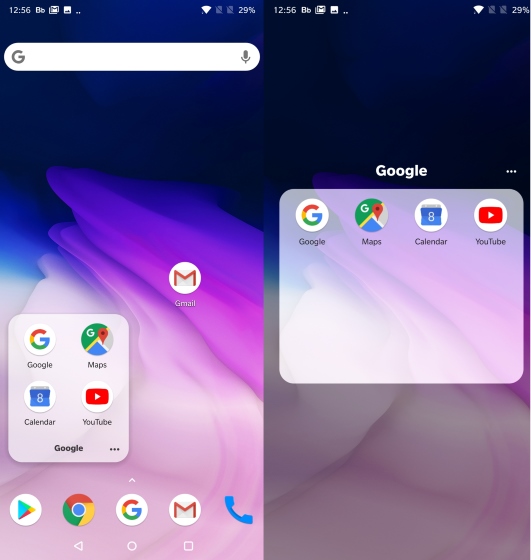This image displays two side-by-side screenshots of a smartphone's homepage, capturing subtle yet distinct differences. Both screenshots feature an almost identical colorful background. The left background showcases a vivid pink and purple swirl reminiscent of oil and water patterns, merging upwards and to the left before fading into a darker blue area. The right background uses the same image but is toned down, presenting a darker, less vibrant version.

At the top of both screens, the time reads 12:56. The status bar includes two overlaid white envelope icons, a white photo icon, two white dots, a full Wi-Fi signal icon, and a battery indicator showing 29%. On both screens, a white search bar is positioned left of center, adorned with a gray "G" logo on the left and a gray microphone icon on the right.

Below the search bar on the left screen, various apps are dispersed. Among them is a single Gmail icon. A prominent white translucent rectangle contains four app icons: Google, Maps, Calendar, and YouTube, with the text label "Google" displayed in black beneath the icons. The bottom row of apps includes the Play Store, Chrome, Google, Gmail, and a blue phone icon.

In contrast, the right screen contains a single white translucent rectangle labeled "Google" in white text, accompanied by three white dots to its right. Inside this rectangle are the same four app icons: Google, Maps, Calendar, and YouTube, maintaining consistency in app organization but differing in visual presentation.

Overall, this detailed comparison highlights the nuanced variations between the two displayed homepages, emphasizing differences in background vibrancy and app layout.